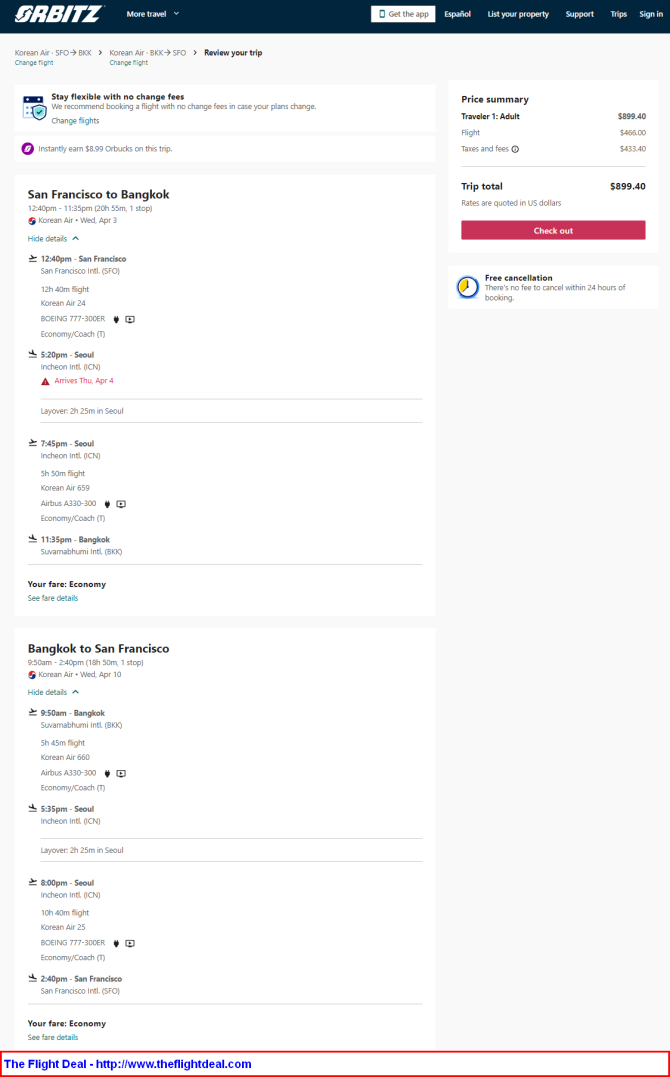A screenshot of a user's computer screen showcasing the Orbits website. At the top of the screen, the word "Orbits" is prominently displayed in white text within a full-width black rectangle. The top navigation bar includes various options such as "More Travel," "Get the App," "Espanol," "List Your Property," "Trips," "Support," and "Sign In."

Below the navigation bar, a banner highlights the flexibility of travel options, noting "Stay flexible with no change fees." Further down, details of a specific flight itinerary are visible, including a route from San Francisco to Bangkok. Small airplane icons are used to denote travel segments, with mentions of layovers and durations for each leg of the journey.

The itinerary and flight deal information are derived from a website, "http://www.theflightdeal.com," which is rendered in clickable blue text. This section is outlined by a distinct red rectangle. The cost of the highlighted flight is prominently displayed at the top, amounting to $899.40.